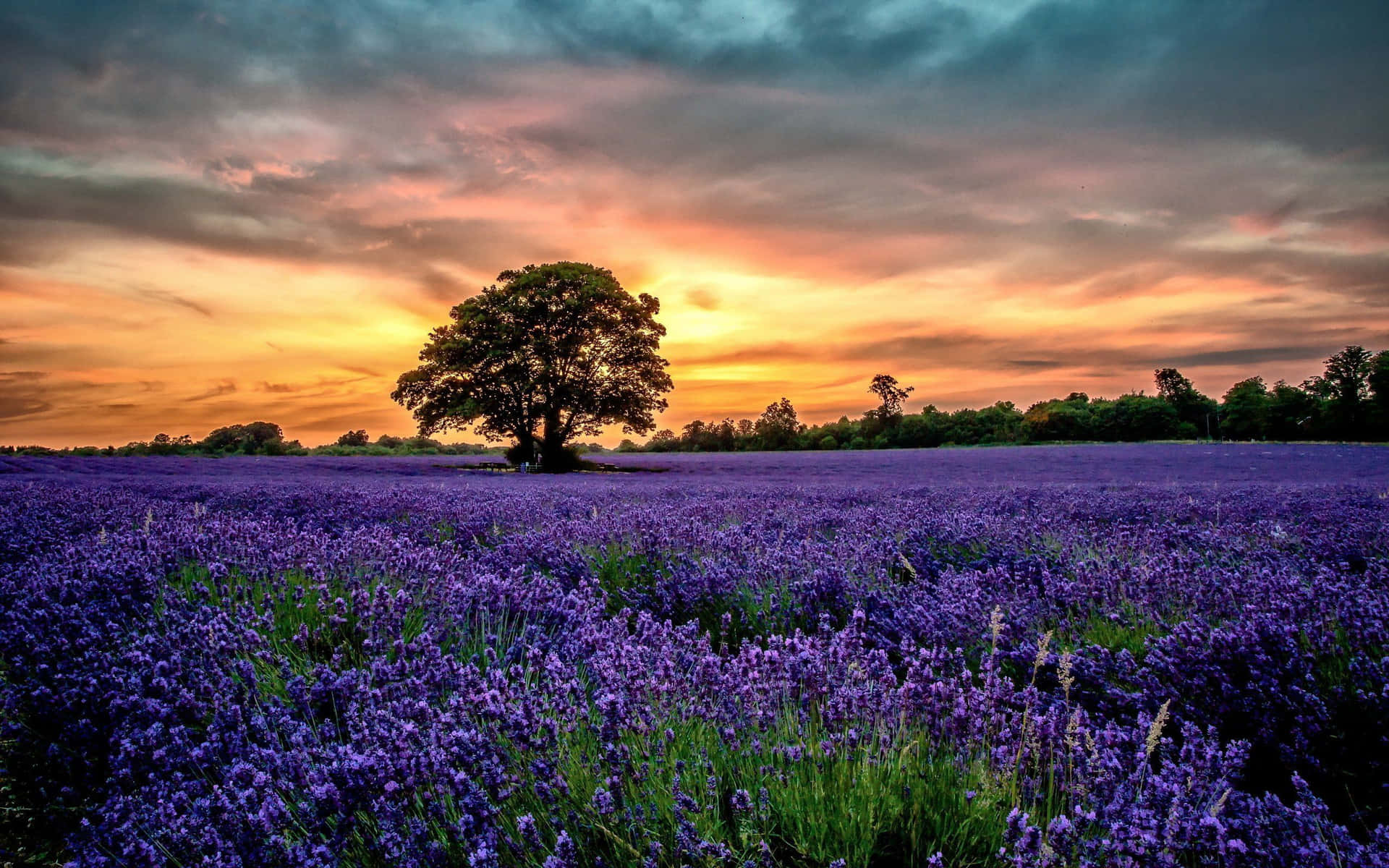This professional-quality photograph captures the serene beauty of nature during sunset. The image presents a breathtaking field of purple flowers that resemble lavender, extending towards a distant tree line. Dominating the center of the frame is a solitary, lush tree with a full canopy of leaves. The sky above displays a mesmerizing gradient, transitioning from deep blue at the top through bands of gray clouds tinged with pink and light blue, down to an orange and yellowish glow near the horizon. The backdrop of green trees lines the horizon, adding depth to the scene. This detailed composition offers a ground-level side view, where the purple flowers intermingle with hints of green foliage, creating a picturesque landscape suffused with the warm and tranquil hues of the setting sun.